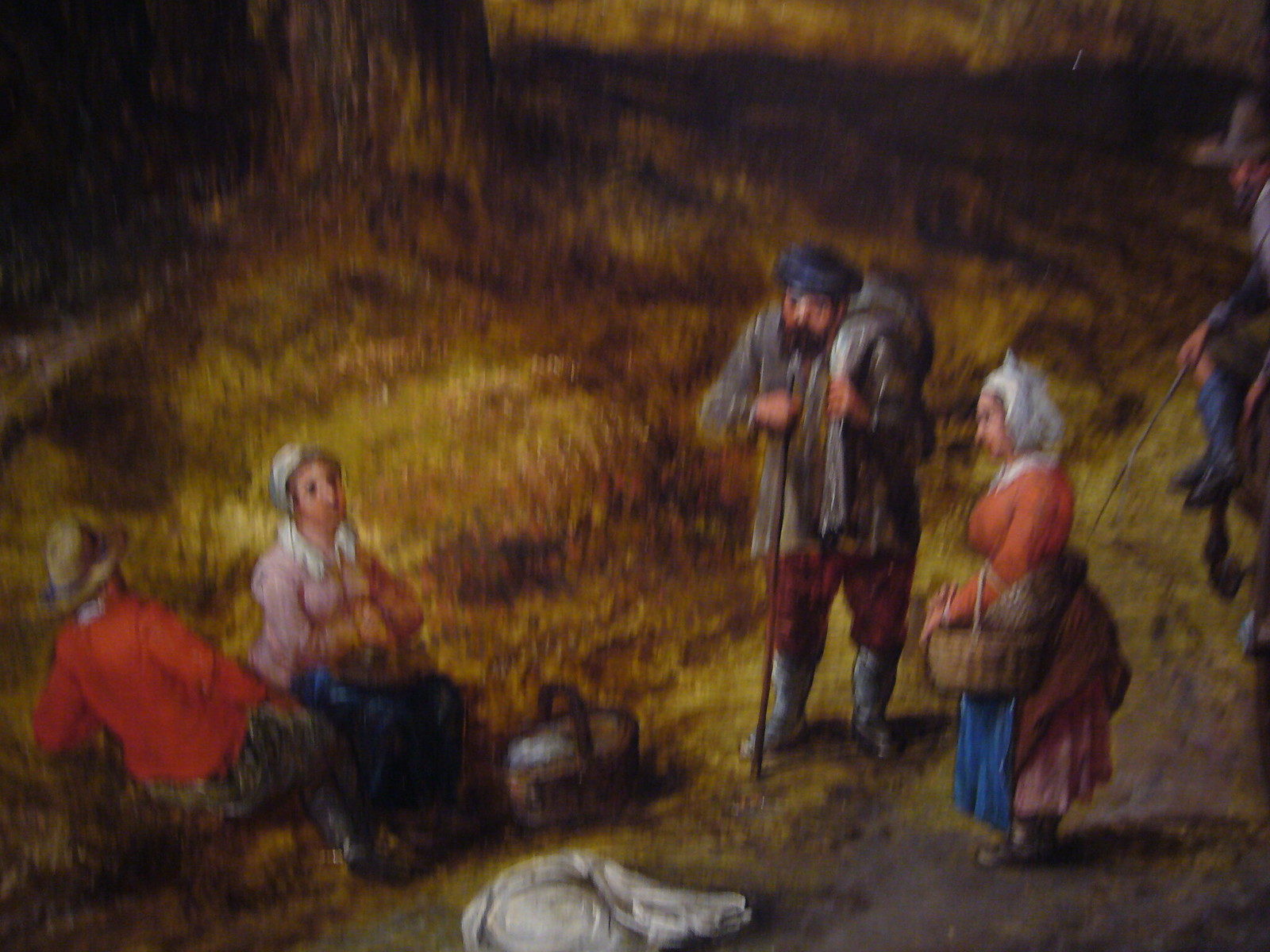This slightly blurry, horizontal oil painting captures a group of old pioneer-type people outdoors in a forest with a yellow grass environment. Central to the composition is a bearded man, stocky in build, wearing big gray boots, red pants, and a grayish-brown jacket, with a blue rolled-up hat on his head. He holds a walking stick in one hand and possibly a bag or an animal draped over his left shoulder. Beside him stands a woman in a blue dress with an orange-salmon blouse with a white collar, and a traditional white bonnet. She holds a picnic basket along with another basket on her arm.

To the left, two seated figures capture attention: a man in an orangish-red shirt and green or camouflage-style pants, wearing a traditional straw hat, and a woman in a pink blouse with a white collar and a white bonnet. Beside them lies an old traditional thatch picnic basket and a white towel or blanket spread on the ground. 

In the background, to the right of the central figures, another man, partially obscured and wearing what appears to be a cowboy or another straw hat, is visible; he is dressed in blue boots. The entire scene feels imbued with a nostalgic, old-timey atmosphere, reinforced by the traditional garments and serene outdoor setting.